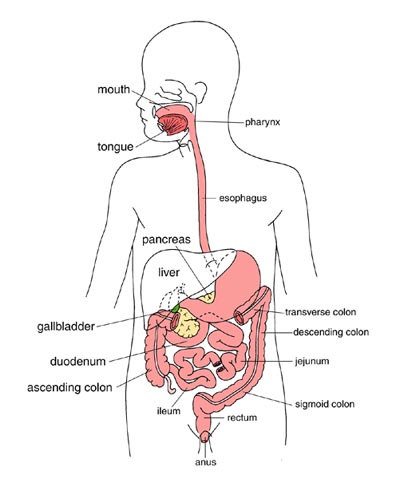The image is a detailed colored pencil illustration of the human digestive system within a black-bordered, white-outlined human figure. The person is facing to the left, and while the eyes are not visible, several internal organs are meticulously drawn and labeled. The digestive tract is the focus, depicted in various colors with predominance of pinkish-red hues, and accented by yellow and green shades for different organs. Starting from the top, the illustration features the mouth and dark pink tongue, leading down to the pharynx and pink esophagus, which extends into the chest area. The liver and pancreas are shaded in black and white, while the gallbladder and ascending colon are also illustrated in distinct colors. The image continues to show the stomach and intestines, highlighting the duodenum, jejunum, ileum, descending colon, transverse colon, and sigmoid colon. At the very base of the illustration, the rectum and anus are clearly depicted. Labels in black lettering identify each part, including the limb, ensuring a comprehensive visual guide to the human digestive system.